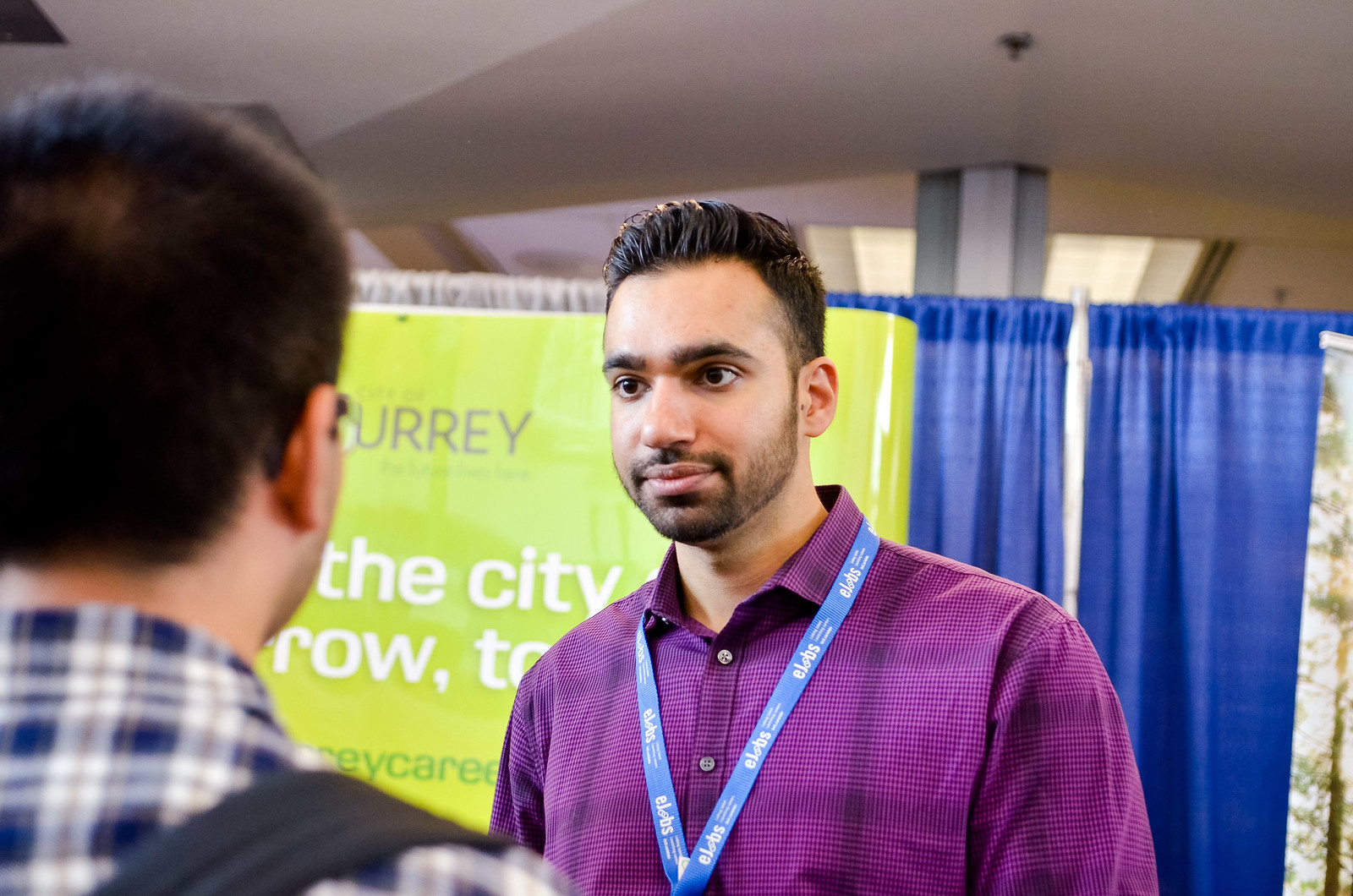This photograph captures a moment at what appears to be a convention, distinguished by the typical convention-style curtains used to separate spaces. The background features a fluorescent green backdrop with partially obscured text, including the word "Surrey" and a phrase beginning with "the city," though it's blocked by the two men in the foreground. The man facing the camera on the right is of East Indian descent, sporting a short dark hairstyle, light facial hair, and wearing a purple button-down shirt, complemented by a blue lanyard around his neck. He appears to be intently listening to the man on his left. The other man, whose back is to the camera, has dark hair, wears glasses, and dons a blue and white plaid shirt. Their conversation is set against a backdrop of blue and white curtains, a ceiling, and a support post, encapsulating a typical convention dialogue setting.